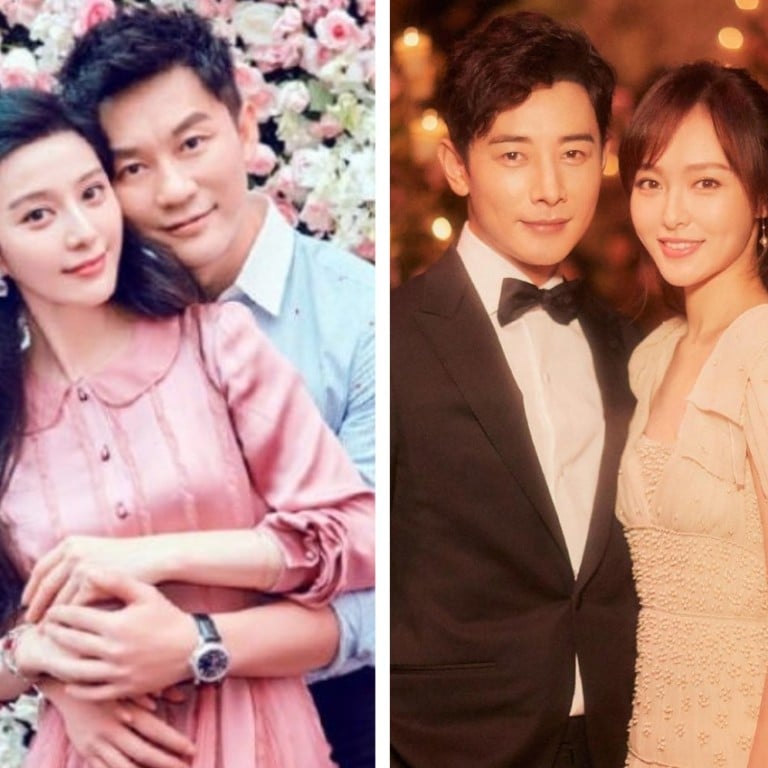In these two side-by-side photos, we see what appears to be the same Asian couple in different settings. The left image features the woman in a pink dress with a rounded, fold-down collar, standing next to a man in a blue dress shirt with a white collar and dark pants. The man, who has slightly spiky hair and is wearing a black watch, has his arm wrapped around her. Both are standing in front of a vibrant backdrop filled with pink and white roses. In the right photo, the woman stands to the right, now adorned with beaded earrings and a glamorous, beaded, cream-colored dress. The man stands on her left, dressed in a sharp white dress shirt, black suit, and black bow tie, smiling. The background of this second photo is blurred, emphasizing their formal attire.